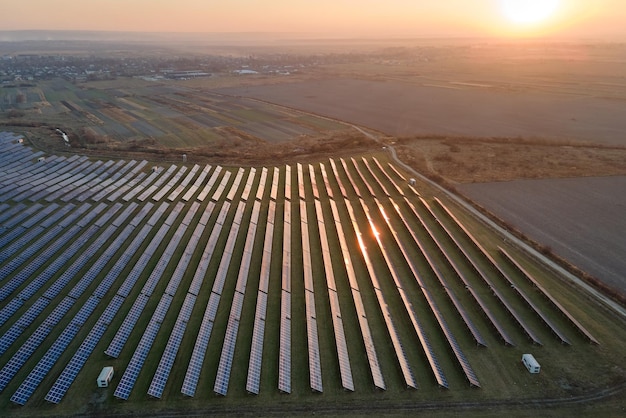The image captures an aerial view of a vast solar farm during sundown. The scene features extensive rows of solar panels meticulously lined up across a flat, desert-like landscape. These rows stretch out beyond the frame, indicating the expansive scale of the solar array. In the upper right-hand corner, a brilliant sun sets, casting an orange and yellow hue across the sky. Toward the left of the image, a small town or cluster of buildings is faintly visible, situated beyond a road that runs adjacent to the solar panels. The background fades into barren dirt plains interspersed with scrub oak and weeds, while a couple of white, rectangular structures, possibly mobile homes or large trucks, are scattered among the panels. The overall focus remains on the immense field of solar panels, designed to harness solar energy, which are now bathed in the waning light of the setting sun.